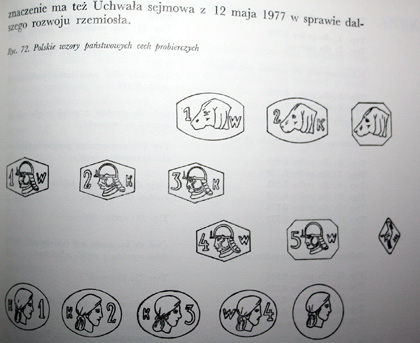The image depicts a black-and-white page from what appears to be an educational or coloring book for children, written in Polish. The layout features a series of line drawings that resemble coins or stamps, each adorned with distinct images such as animal heads, a soldier in a helmet, and a woman’s face in profile. These sketches are numbered 1 through 5 and are outlined in various shapes like ovals and hexagons. Above these illustrations, there is Polish text that includes the date "12 May 1977" and possibly references a SEJM resolution or a publication related to craft development, indicated by the smaller text "72." The entire page is printed with black ink on a white background.